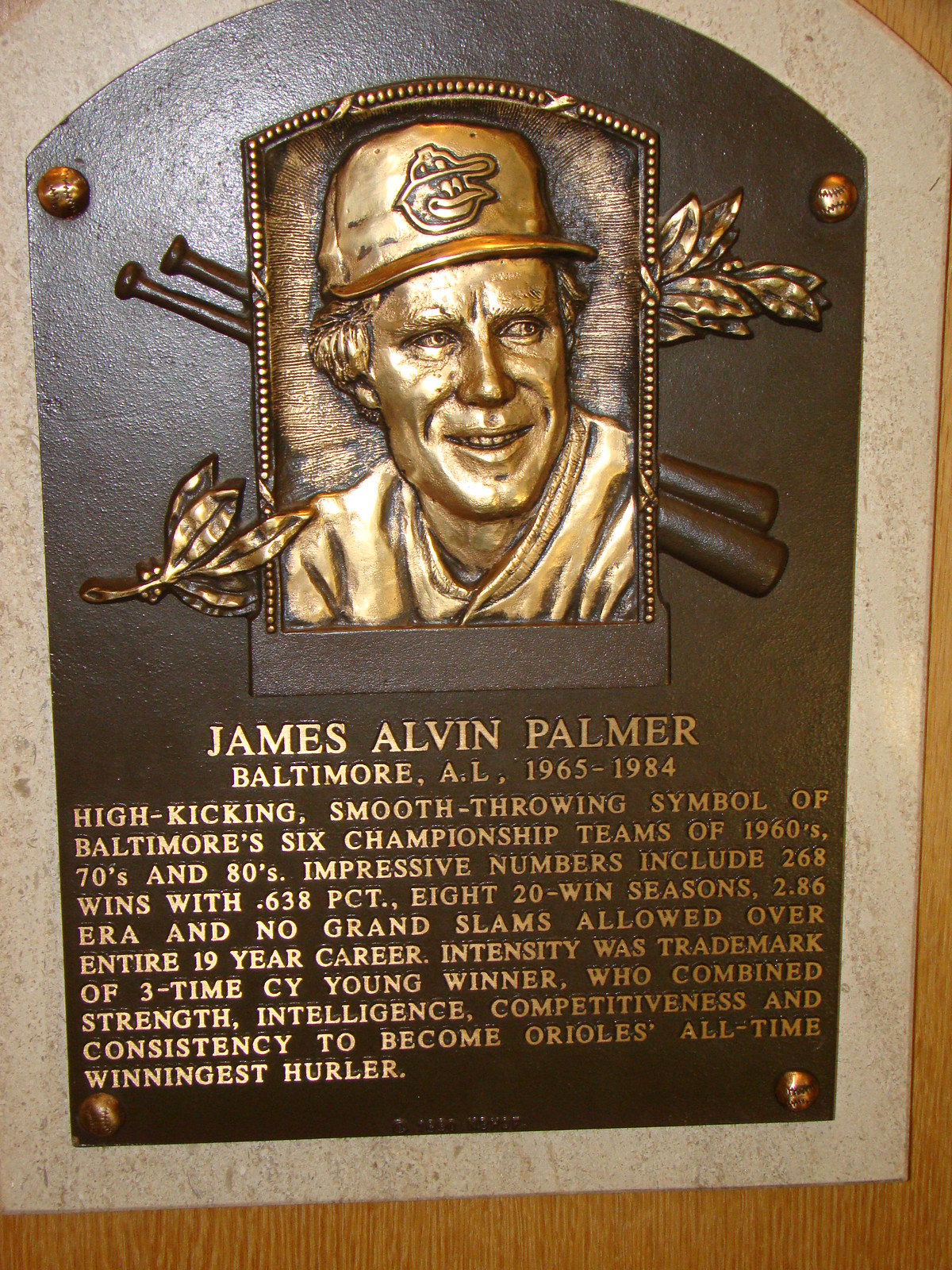The image features a commemorative plaque affixed to a brown wooden wall. The plaque is a dark bronze rectangle with a rounded, beveled top, measuring approximately 6 inches in height and 4 to 5 inches in width. At the top of the plaque, a bronzed, textured relief of a baseball player is prominently displayed. The player is depicted from just below the neck to the top of his cap, wearing a Baltimore Orioles jersey and cap with an Oriole emblem. Behind him are crossed baseball bats and decorative leaves.

Beneath the relief, the text in raised, light-bronze or gold lettering reads: "James Alvin Palmer, Baltimore, A.L. 1965-1984. High-kicking, smooth-throwing symbol of Baltimore's six championship teams of the 1960s, 70s, and 80s. Impressive numbers include 268 wins with a .638 win percentage, 8 20-win seasons, a 2.86 ERA, and no grand slams allowed over an entire 19-year career. Intensity was the trademark of this three-time Cy Young winner who combined strength, intelligence, competitiveness, and consistency to become the Orioles' all-time winningest hurler."

This detailed tribute possibly resides in the Baseball Hall of Fame, at Jim Palmer's birthplace, or in a museum honoring the storied legacy of this revered Baltimore Orioles pitcher.